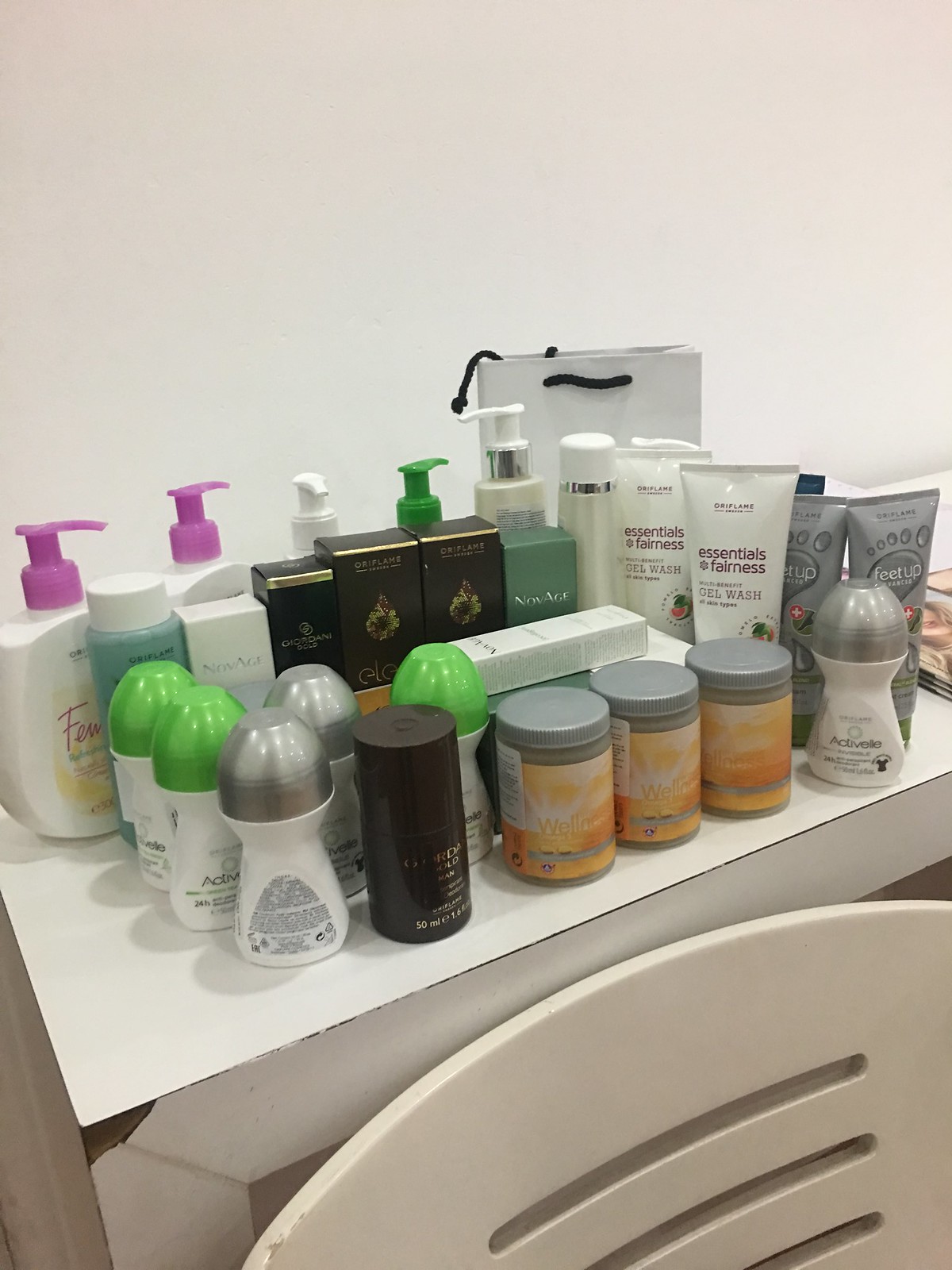This photograph captures a neatly arranged countertop, either in a bathroom or a store, filled with a variety of bath and cosmetic supplies. The countertop, constructed from white wood, matches the pristine white wall in the background, enhancing the clean and orderly appearance. At the bottom of the image, the top of a white wooden chair is partially visible, positioned in front of the counter.

The assortment of products on the counter is visually striking, with items varying in shape and color, predominantly featuring shades of gray, green, black, and teal. Among these, there are four lotion containers at the back, two of which are distinguished by their purple nozzles. In the foreground, three identical plastic jars with orange labels stand out. The diverse collection includes items that appear to be gel washes, foot care products, deodorants, and various other items packaged in cardboard boxes. Each product is displayed in an organized manner, making the countertop both functional and aesthetically pleasing.